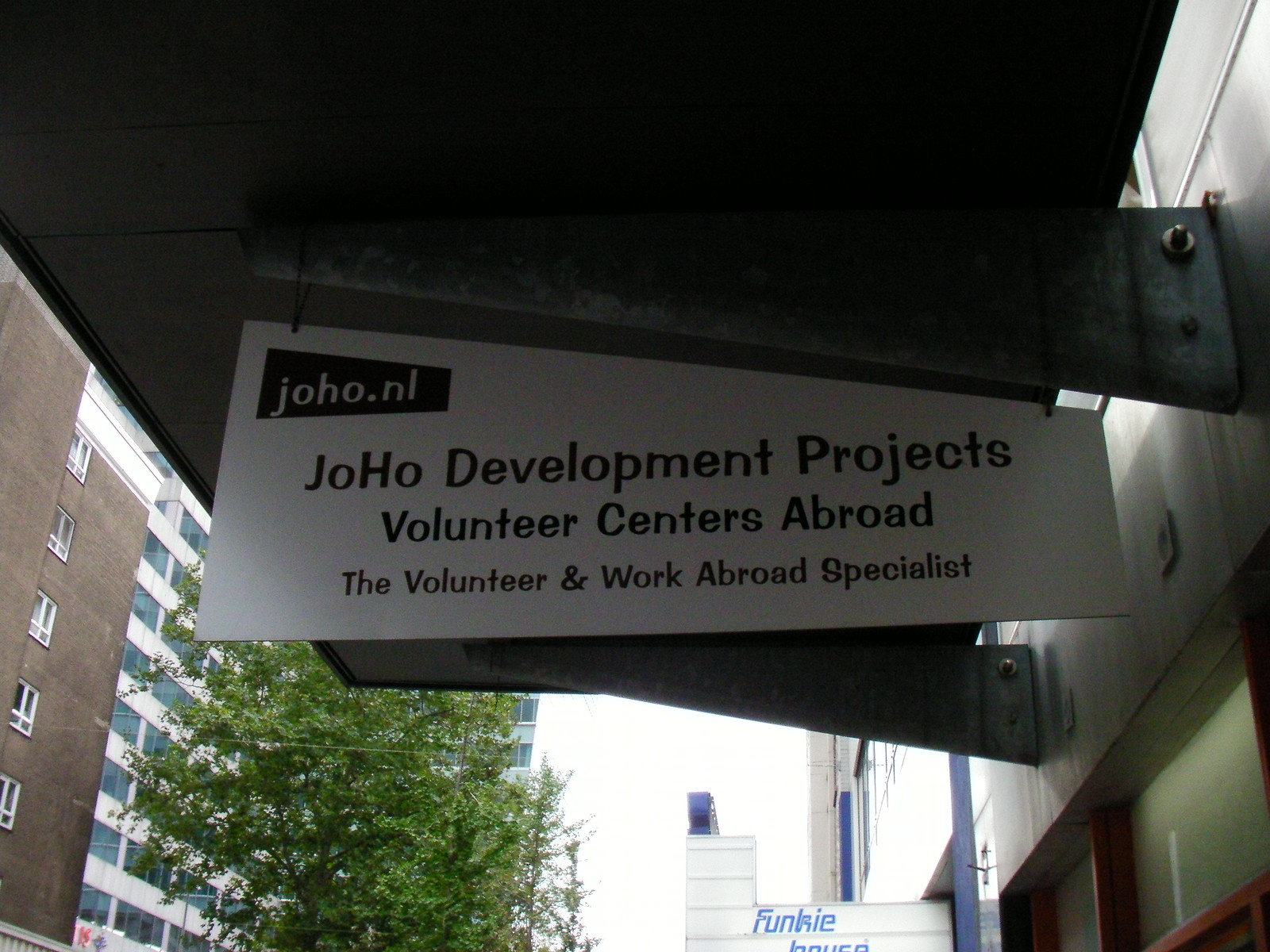The image captures a busy urban scene featuring a somewhat worn-out building with a metal overhang partially shading a prominent sign for Joho Development Projects, located on the right side of the street. The overhang appears to provide shelter from weather elements, extending from the building's facade above the sidewalk. The focal point of the photo is a white sign with black text, announcing "Joho Development Projects, Volunteer Centers Abroad, the Volunteer and Work Abroad Specialist." In the upper left corner of the sign is the Joho NL website, displayed in white text on a black background. The backdrop includes tall buildings with varying facades, including a white office building with blue windows and a red brick building with white windows. Trees are interspersed along the street, and additional billboards and signs, such as one displaying "Funky" in blue text, can be seen in the distance, enhancing the vibrant, layered cityscape.